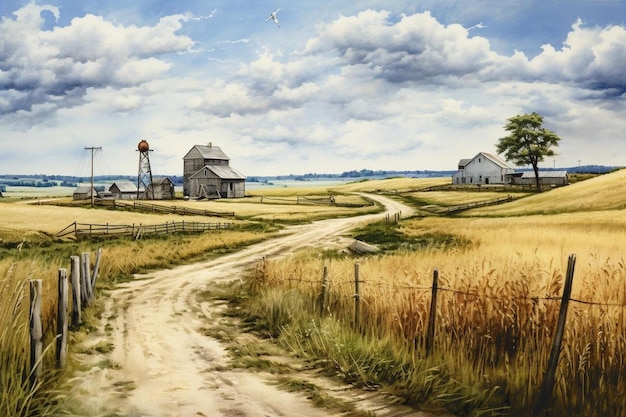This detailed painting or AI rendering depicts a serene countryside scene featuring a long, unpaved, and curving dirt road bordered by wooden fence posts connected with wire. On either side of the road lies a grassy field with golden hues. In the distance to the right, a white farmhouse stands tall beside a larger tree. On the left side, there are several gray farm buildings, including a potential water tower, and a power pole. There are a total of six structures on the left and two on the right, with the road winding between them. Smaller trees dot the distant background under a blue sky filled with white clouds, adding to the tranquil atmosphere of this rural setting.